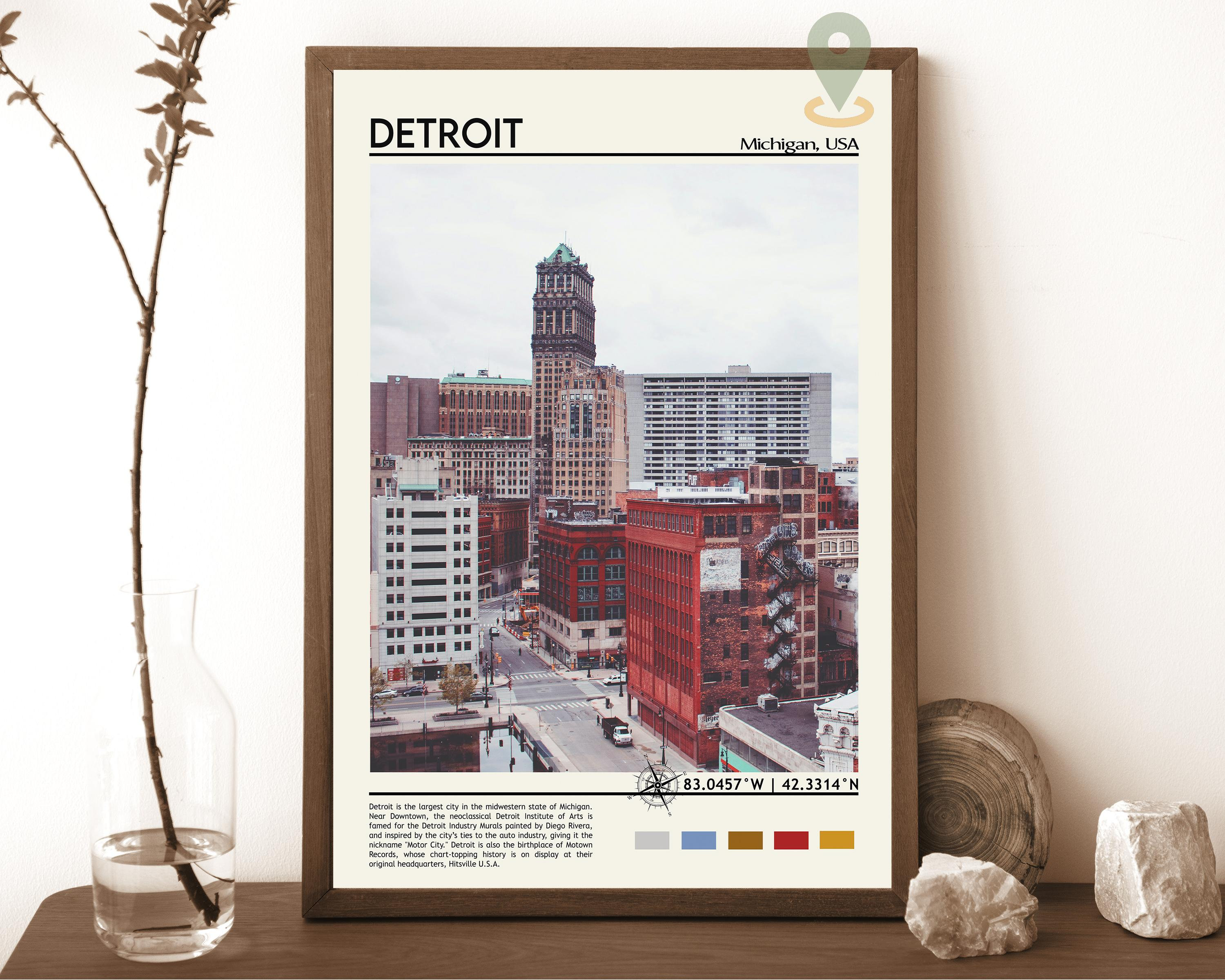This is a rectangular landscape photograph capturing a small dark brown wooden shelf. Prominently displayed on the shelf is a large framed painting that features a cityscape with towering skyscrapers and prominently displays the word "Detroit." The painting itself is encased in a wooden frame that complements the shelf. On the right side of the shelf, there are three large, smooth rocks arranged neatly. On the left side, a small glass vase filled with water houses a plant. The plant, predominantly brown, has a few green leaves sprouting at the top, adding a touch of life and contrast to the scene. The overall composition of the photograph showcases a harmonious blend of art, nature, and natural materials.